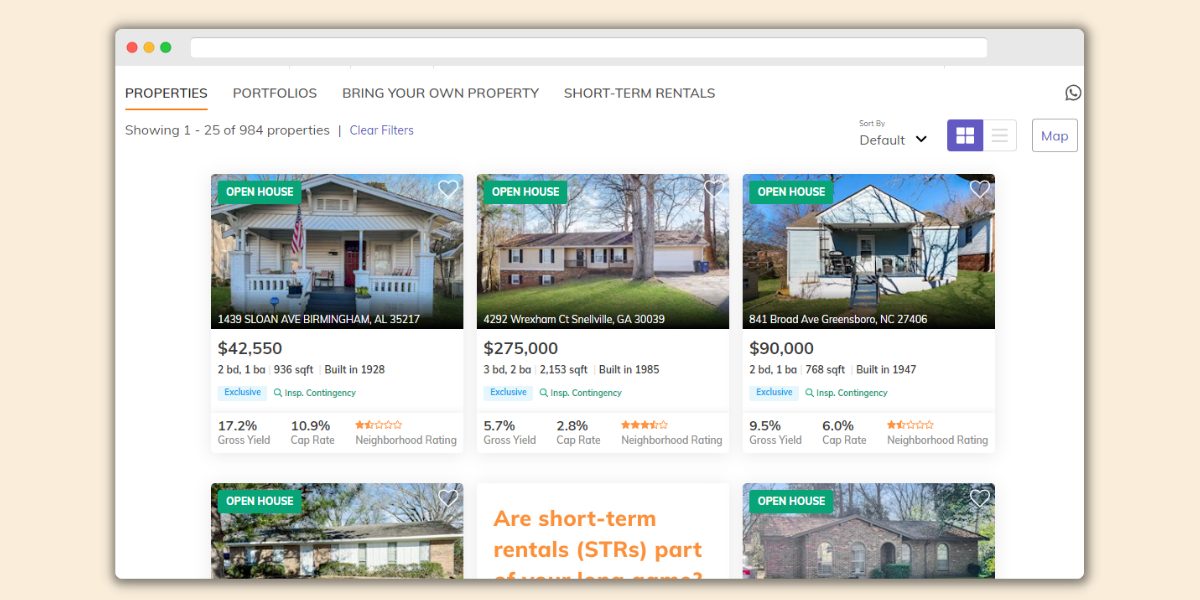This image is a detailed screenshot from a real estate website showcasing various properties for sale. The properties are displayed with their respective prices: $275,000, $90,000, and $42,550. Each property image prominently features an 'Open House' notification in the top left corner. Below the images, performance metrics such as cap rate and gross yield are listed, alongside neighborhood ratings presented in a 5-star format. 

At the very top of the webpage, there is a navigation menu with several options: "Properties," "Portfolios," "Bring Your Own Property," and "Short Term Rentals." Directly above this menu is a white search bar, flanked on the left by three horizontal, colored circles—red, yellow, and green. The page is set against a white background, providing a clean and uncluttered appearance. 

On the top right, users have the option to sort the listings. There's also a button and a key icon to switch the display mode to a map view.